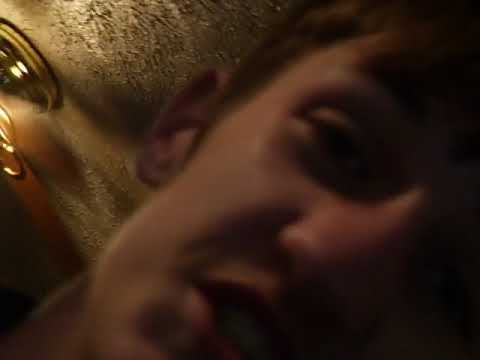The image is a very blurry and grainy close-up selfie of a teenage boy with pale skin. His face, which has large ears and short brownish-orange hair, is extremely close to the camera, taking up about 60% of the frame and tilting to the right. His mouth is slightly open, revealing his teeth, though the eyes are almost indistinguishable due to the shadowy conditions. The background, visible only in the upper left corner, features a dimly lit scene that appears to be a painted house with an orange porch lamp. The background elements also suggest a yellowish or off-white ceiling, potentially with a ceiling fan or light fixture, adding to the overall blur and graininess of the image. Overall, the photo seems like an accidental capture in a dark setting, reflecting both the person and the indistinct surroundings.